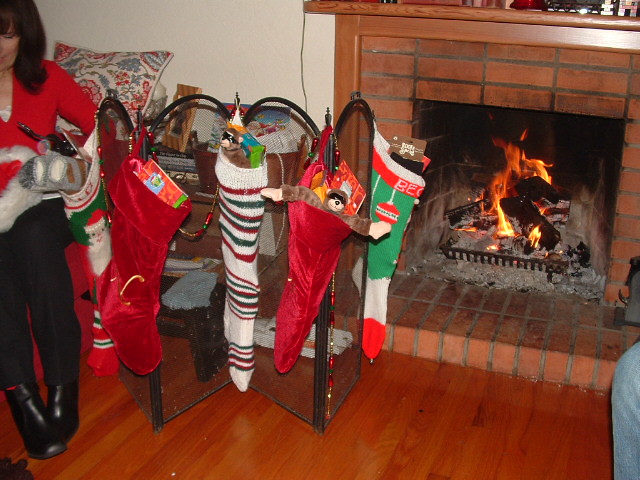This color photograph captures a cozy, festive living room scene centered around a vibrant, blazing fireplace. The fireplace, built with brown bricks and topped with a matching wooden mantle, bathes the room in a warm glow. Gray ash and charcoal rest at the hearth, evidence of a long-burning fire. To the right of the fireplace is a black metal grate guard, standing next to it rather than in front.

Adorning this guard are five Christmas stockings, each uniquely decorated: a green one with a Santa design, a plain red velvet one, a red-and-green striped white stocking, another red velvet one, and a white stocking with a green section featuring ornaments, finished with red accents. These stockings are filled with small toys peeking out, adding to the festive atmosphere.

The glossy, diagonal hardwood floor beneath the fireplace and stockings enhances the room's warmth with its bright orange hue. On the far left of the image, partially visible, sits a woman dressed in holiday attire—a red V-neck shirt paired with black pants and boots. Her shoulder-length brown hair curls softly at the ends. Behind her rests a white pillow adorned with a woven red and blue floral design. Just barely visible in the bottom corner of the right side of the image is the edge of another person's knee, clad in blue jeans, hinting at the presence of more family or friends enjoying this cozy holiday setting.